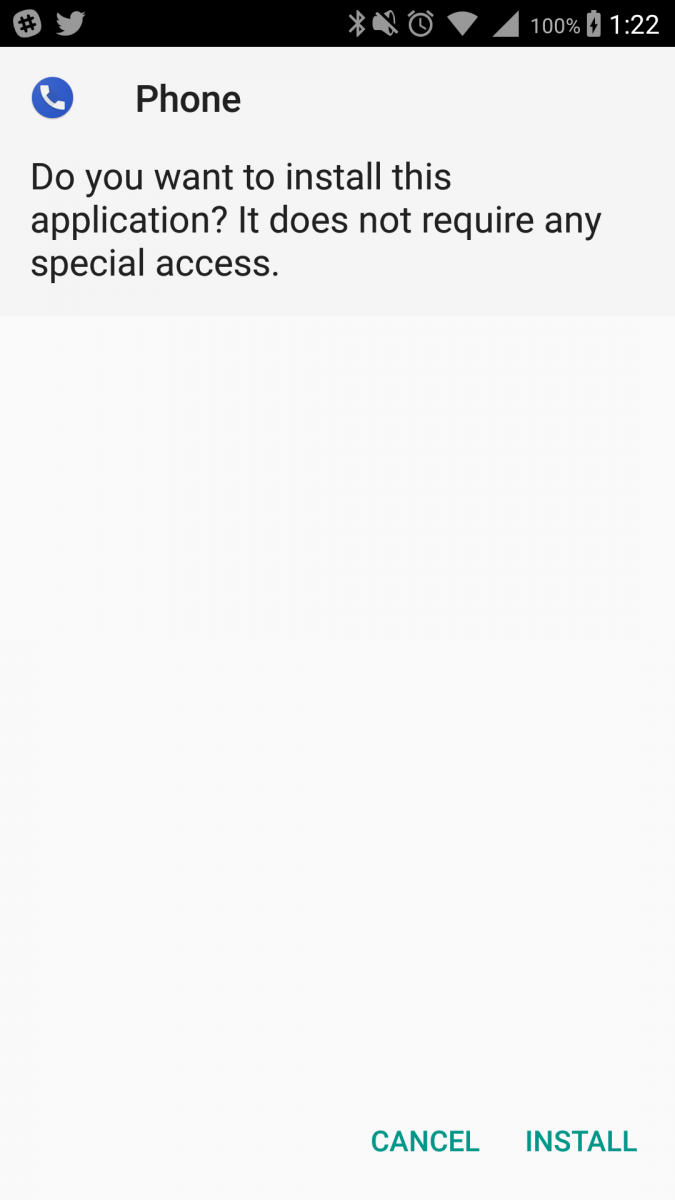This screenshot appears to be taken from a smartphone, likely an Android device, although the specific type of phone is not clearly identifiable due to the lack of borders. The top of the screenshot features a black status bar containing several icons. From left to right, the icons include:
- An icon resembling a tilted hashtag within an almost circular shape
- The Twitter bird logo
- The Bluetooth icon
- A sound icon with a crossing line through it, indicating that sound is muted
- A clock icon
- A filled Wi-Fi icon indicating a strong connection
- A filled cellular signal icon also indicating full reception
- The text "100%" suggesting full signal strength
- A fully charged battery icon with a lightning bolt, indicating the phone is charging
- The time "1:22"

Beneath the status bar, on the left side, there is a blue circle with a white phone icon inside it, accompanied by the bolded word "Phone." Immediately below this, there is a gray notification banner reading, "Do you want to install this application?" followed by "It does not require any special access." 

The lower part of the screenshot, in a lighter gray section, presents two buttons for user action: "Cancel" on the left and "Install" on the bottom right.